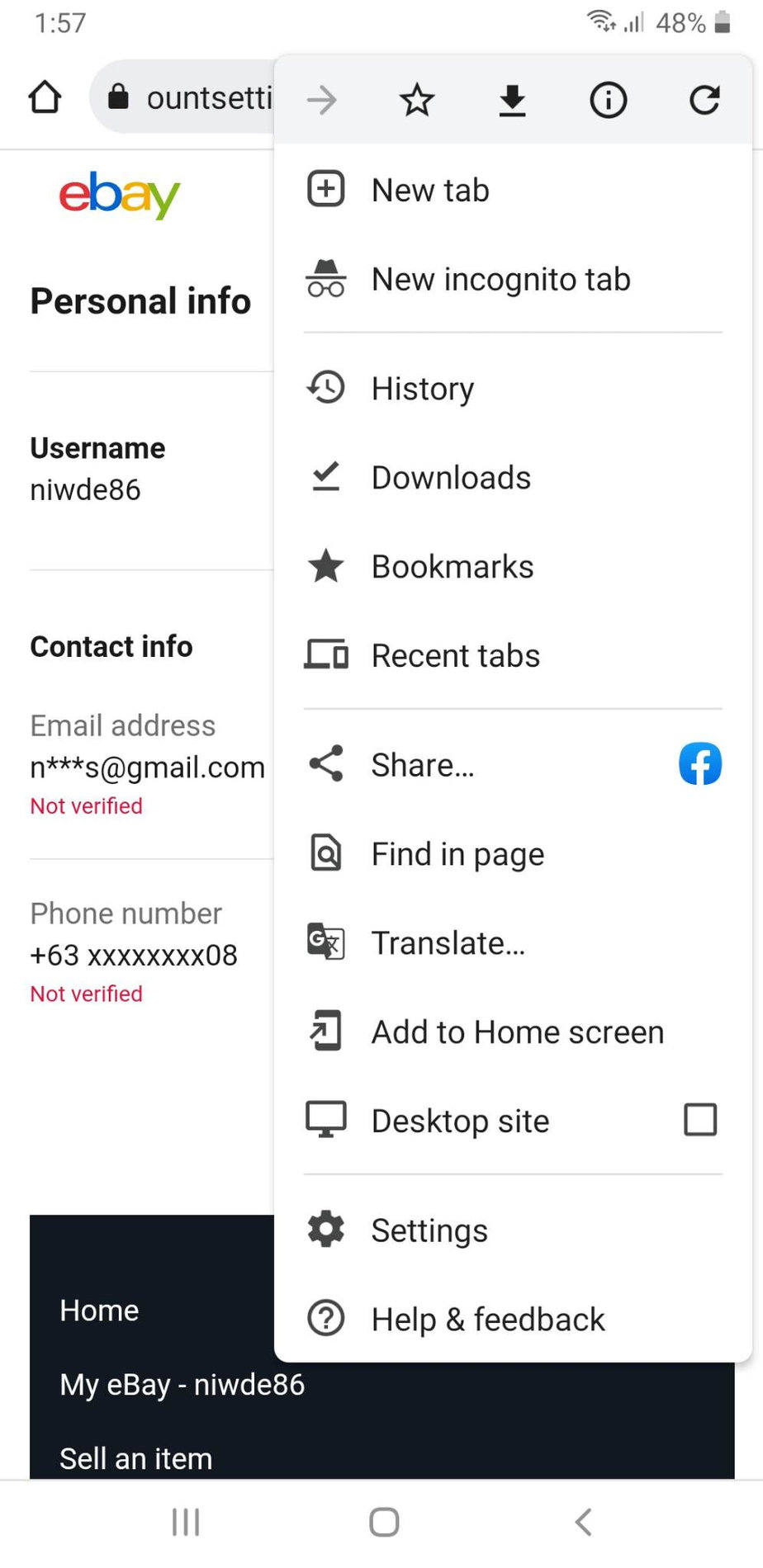This image captures an eBay webpage with a vibrant, multi-colored logo at the top center. The logo letters are distinctively colored: the 'E' in red, 'B' in blue, 'A' in yellow, and 'Y' in green. At the very top of the page, a navigation bar features an account settings icon accompanied by an arrow pointing to the right. There are multiple tabs visible including "New Incognito Tab," "History," "Downloads," "Bookmarks," "Recent Tabs," "Share," "Find in Page," "Translate," "Add to Home Screen," "Desktop Site," "Settings," and "Help & Feedback."

On the left side under the eBay logo, the section is labeled "Personal Info" in black letters. Below this, there is a section displaying the user's username as "NIWDE86," followed by their contact information. Part of the user's email address has been obscured, but it is identifiable as a Gmail address. Similarly, part of their phone number has been redacted, with some digits replaced by X's.

At the bottom of the page, there are clickable icons for navigating through different sections of eBay, including "Home," "My eBay," and "Sell an Item."